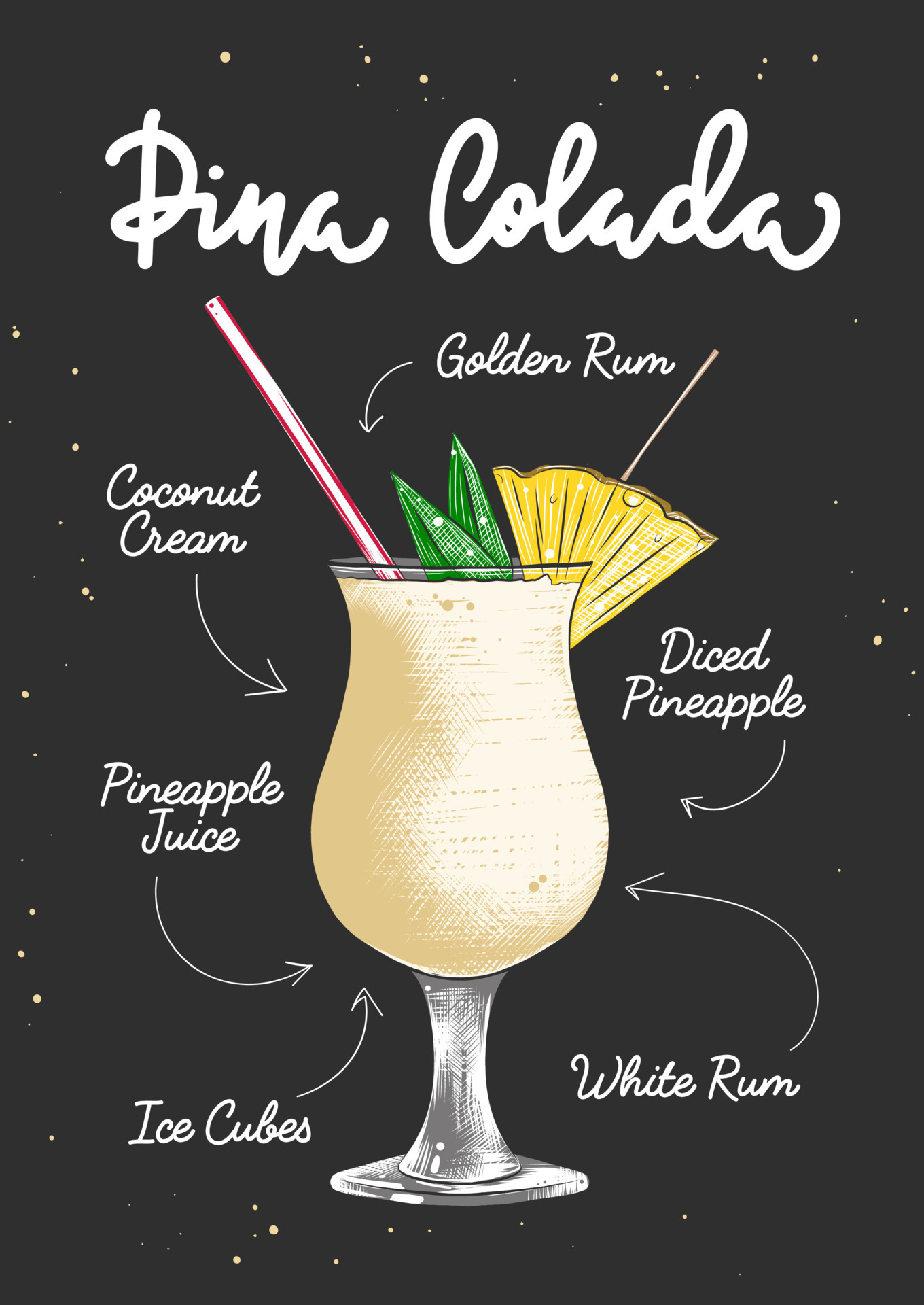The image is a detailed and animated illustration of a piña colada recipe set against a black background speckled with white dots. At the top, the words "Piña Colada" are elegantly handwritten in cursive white font. The centerpiece of the image is a large glass cup containing a creamy white piña colada, garnished with a straw, two pieces of mint, and a slice of pineapple on the rim. Surrounding the glass, arrows point to the various ingredients: golden rum, white rum, coconut cream, pineapple juice, ice cubes, and diced pineapple, each labeled in the same cursive font as the title.